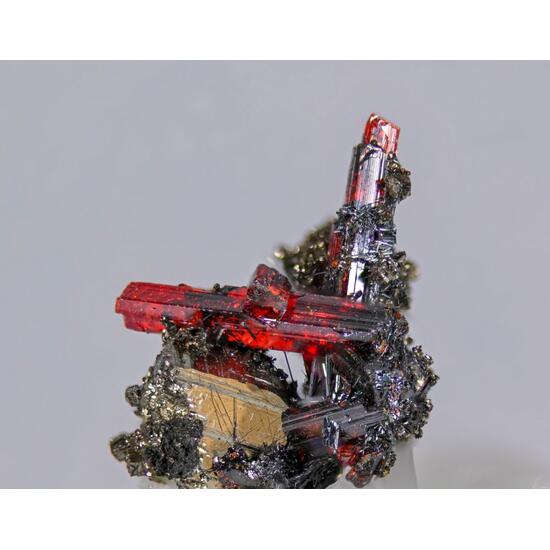The image depicts a complex and captivating mineral formation, dominated by vivid, translucent red crystals that exhibit a primary color intensity with darker, blackish shading adding depth. Surrounding these crystals are metallic, multicolored bismuth-like elements that resemble crystallized patterns often seen in metallic minerals. Some sections have a resemblance to fool's gold or pyrite, contributing to the intricate aesthetics of the formation. Among these crystals, there is a stone that oddly resembles a brick, suggesting a blend of natural and potentially man-made elements. The formation is set against a contrasting gray background, with black charred areas that create a striking visual effect. Alongside, there are additional features including a brown box-like structure and thin red lights, one of which appears melted or distorted, adding to the unique and somewhat enigmatic appearance of the scene.